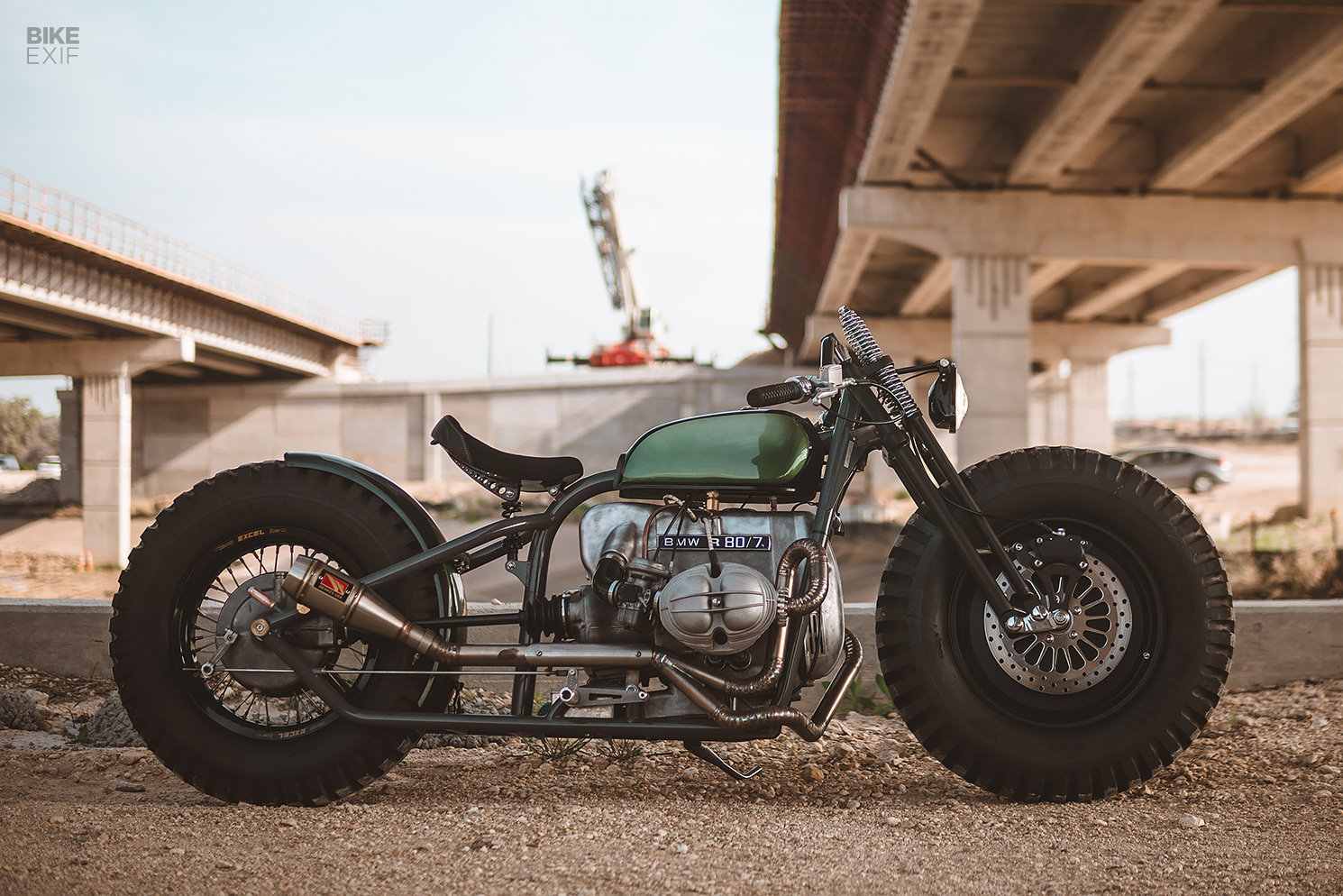The image features a horizontally shot color photograph of a BMW R80/7 motorcycle, prominently displaying a green midsection believed to be the gas tank and labeled with "BMW R80/7." The bike boasts a metallic silver middle section and has large black tires, a black seat, and compact handlebars, sitting very low to the ground. It is parked on a gravel pathway beneath an overpass, with the bridge structure visible in both the upper right and left corners of the image. The background includes a crane-like object near a gray brick wall, some blurred cars, and parts of the freeway system. The sky is bright white, with a hint of blue breaking through. The image credits in the top left-hand corner mention "Bike EXIF."